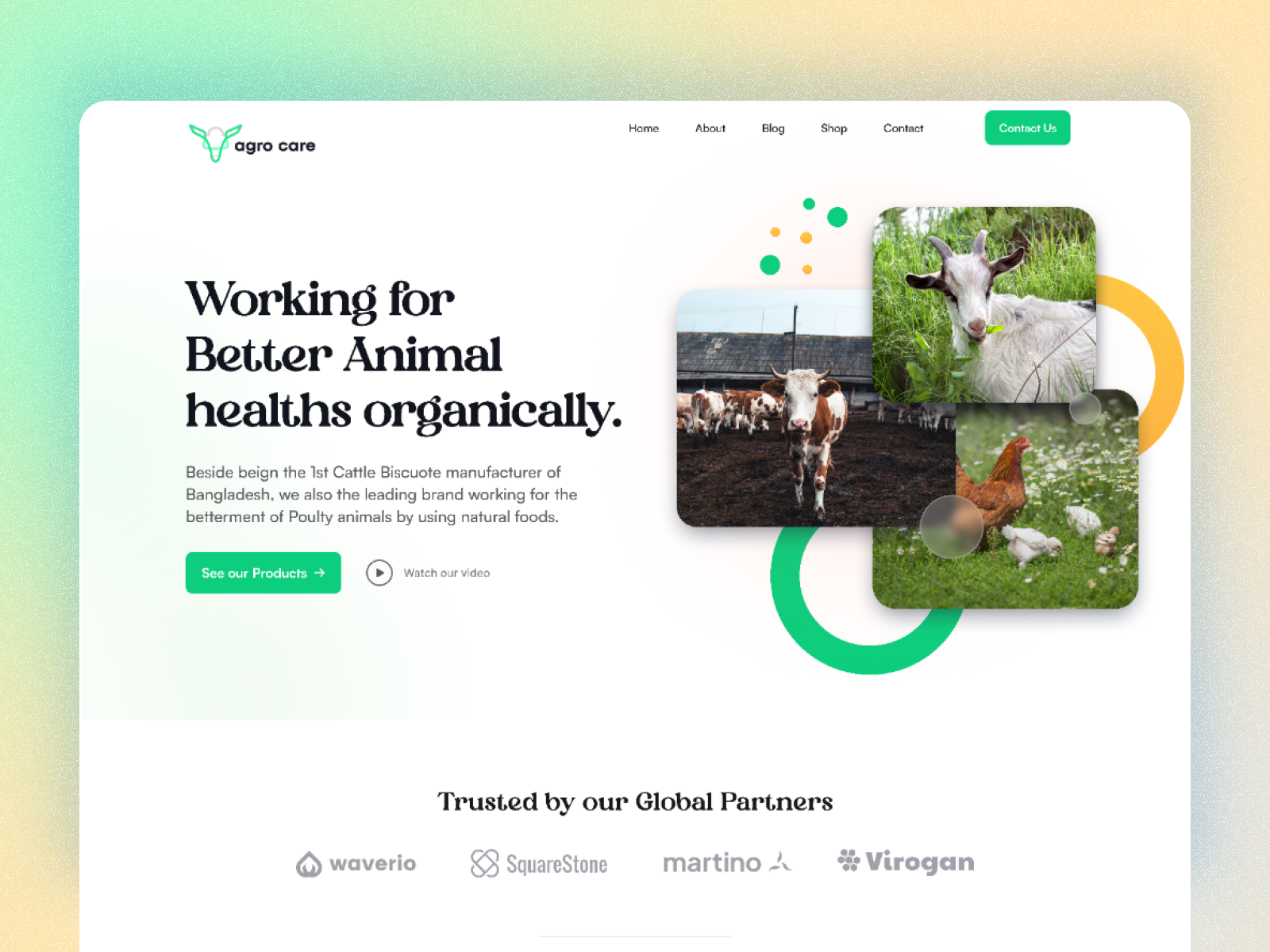This image depicts a web page for Argo Care, displayed on a full computer screen, though the bottom part might be trimmed. The background features a gradient blend with a teal area in the upper left corner, transitioning to a very pale yellow in the lower left corner and upper right section, and to a whitish hue in the bottom right. 

An overlaying white square with rounded corners occupies the center of the page. The website highlights Argo Care's logo, positioned in the upper left corner, next to an animal head icon. Central to the homepage is the text proclaiming, "Working for better animal health organically."

Below this tagline, there are three images depicting different livestock: a cow, a goat, and chickens. An additional message beneath the tagline reads, "Begin the first cattle bisque coat manufacturer of Bangladesh," though it contains a typo ("bisque coat" should be corrected to "basic coat"). Another textual line mentions, "We also, the leading brand," indicating a need for further grammatical editing.

At the bottom of the page, Argo Care emphasizes their global recognition, listing four trusted partners. The company's commitment to animal health, despite some minor English language errors, comes through clearly in this visually appealing web layout.